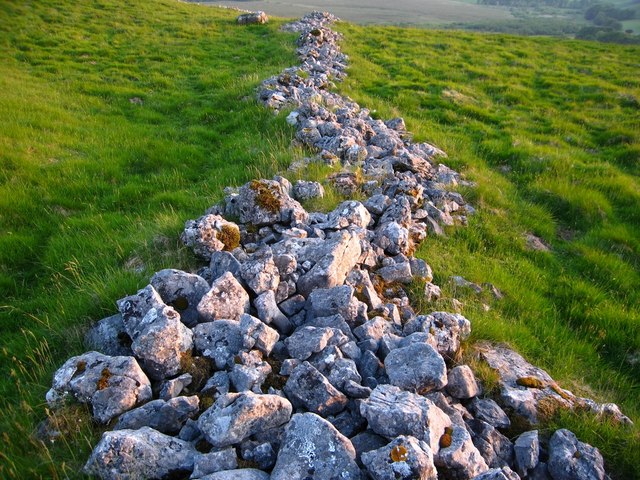The image depicts a lush, green grass-covered hillside in a rural area, with a stunningly vibrant expanse of greenery. Cutting through the center of the photograph from the foreground to the distant horizon, a sinuous path made of medium-sized, light gray stones weaves its way upward. The stone path, which resembles a snake with its slight zigzags and curves, appears to be a man-made formation, possibly serving as a marker or a border dividing the field. The stones are interspersed with patches of brown and green moss, indicating their age and exposure to the elements. In the far distance, at the very top of the photograph, a hint of clouds is visible, accentuating the serene and expansive nature of the landscape.